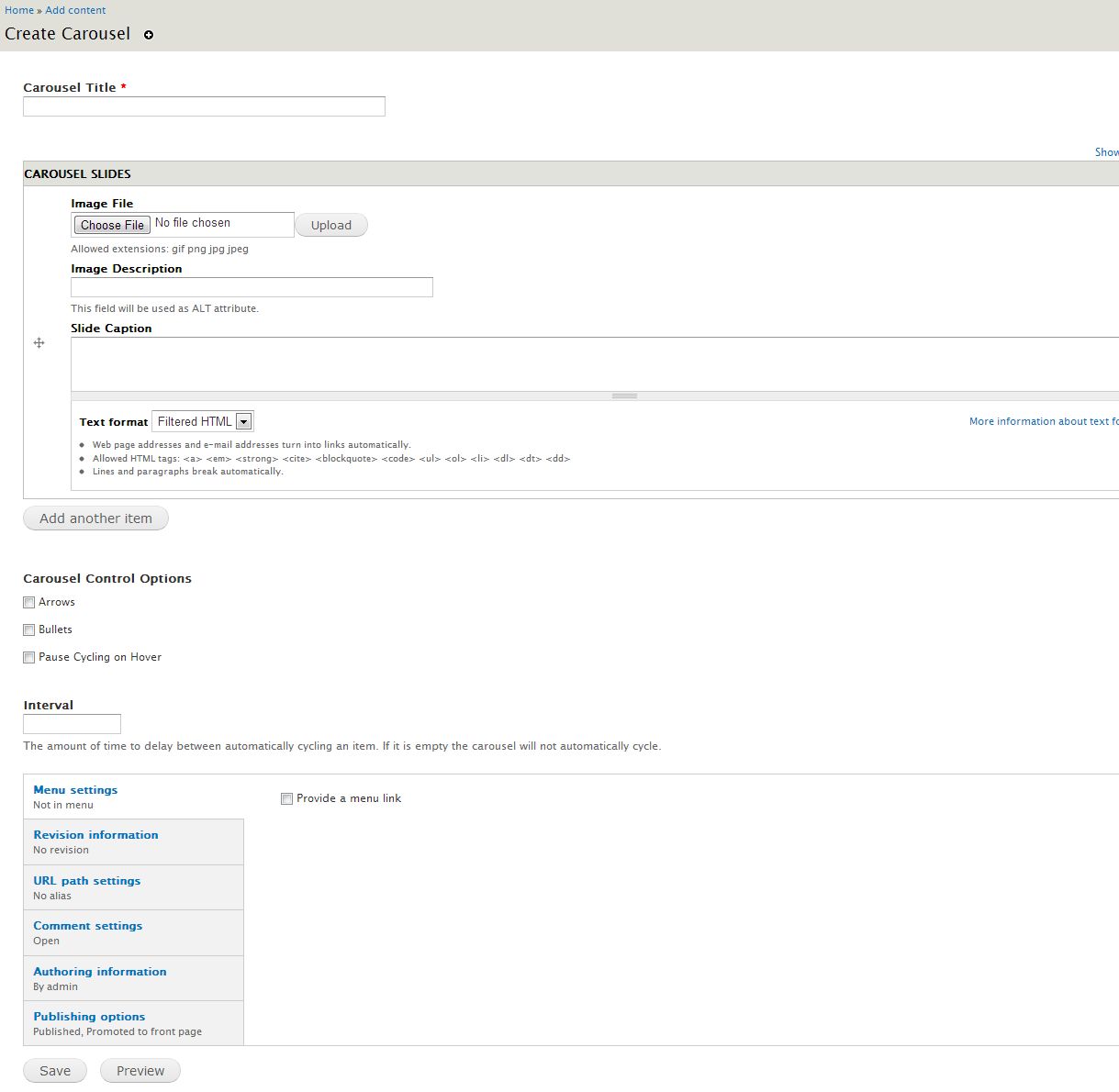Here is a cleaned-up and detailed caption for the image:

---

Screenshot of a web page section titled "Create Carousel." At the top of the section is a white text box labeled "Carousel Title." Below this is the "Carousel Slides" area, which includes several interactive elements. There is a text box for selecting an image file, alongside a "Choose File" button and an "Upload" button. Below the file upload area is a square text box labeled "Image Description," indicating that this will be used in ALT attributes. Further down, there is a "Slide Description" field and a "Slide Caption" field for additional text associated with each slide. At the bottom of this section, there are options for "Carousel Control," including settings for arrows, pagination bullets, and an option to pause cycling on hover.

---